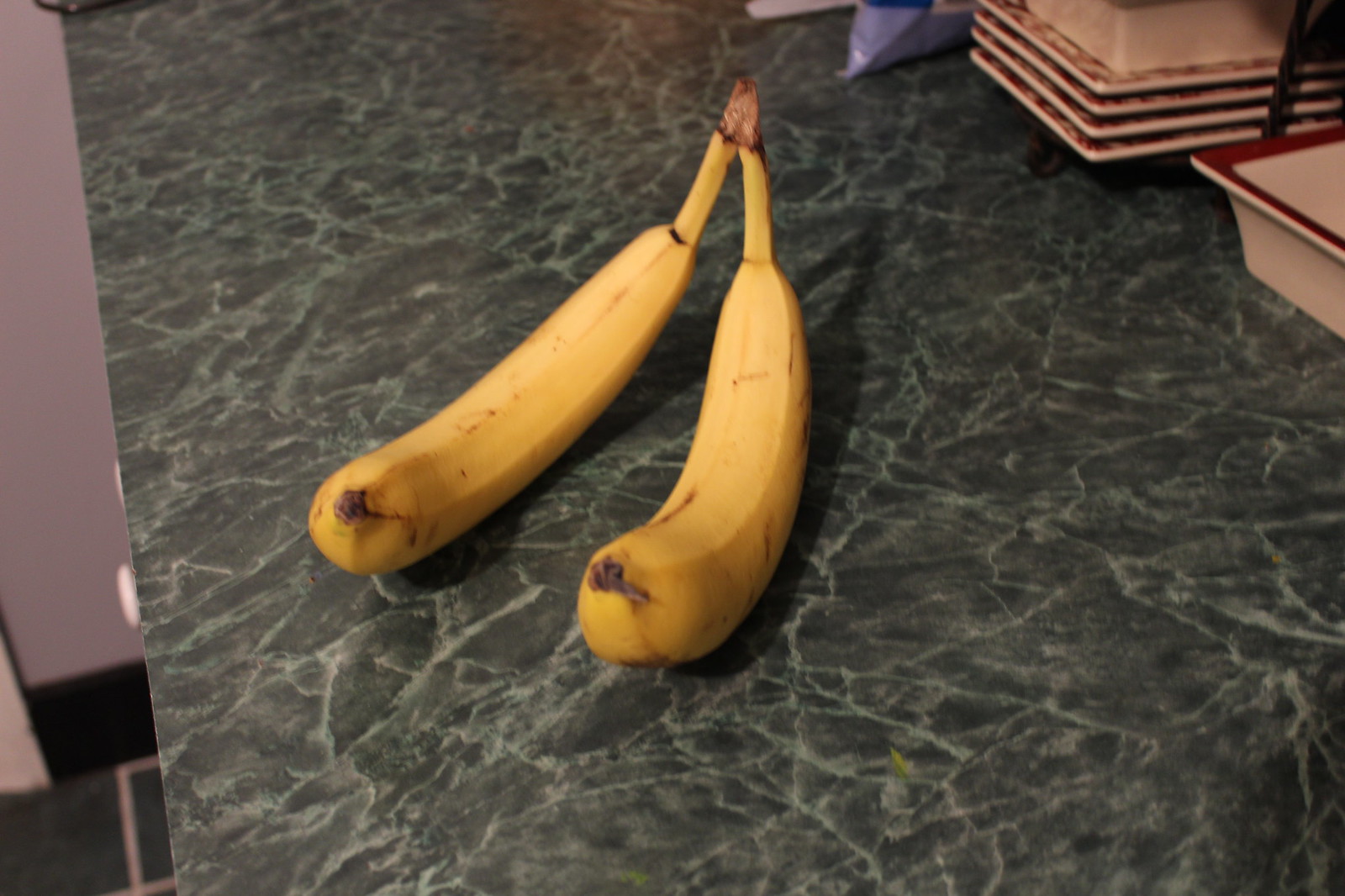Two ripe bananas, with slightly browned ends, are still connected at the stalk and rest on a green counter patterned with white jagged lines resembling marble. Nearby, a partially visible square or rectangular bowl with a red-rimmed lip sits. Scattered around are smaller pieces of chinaware, likely bowls turned upside down, featuring red and white decorations on the underside of the rims.